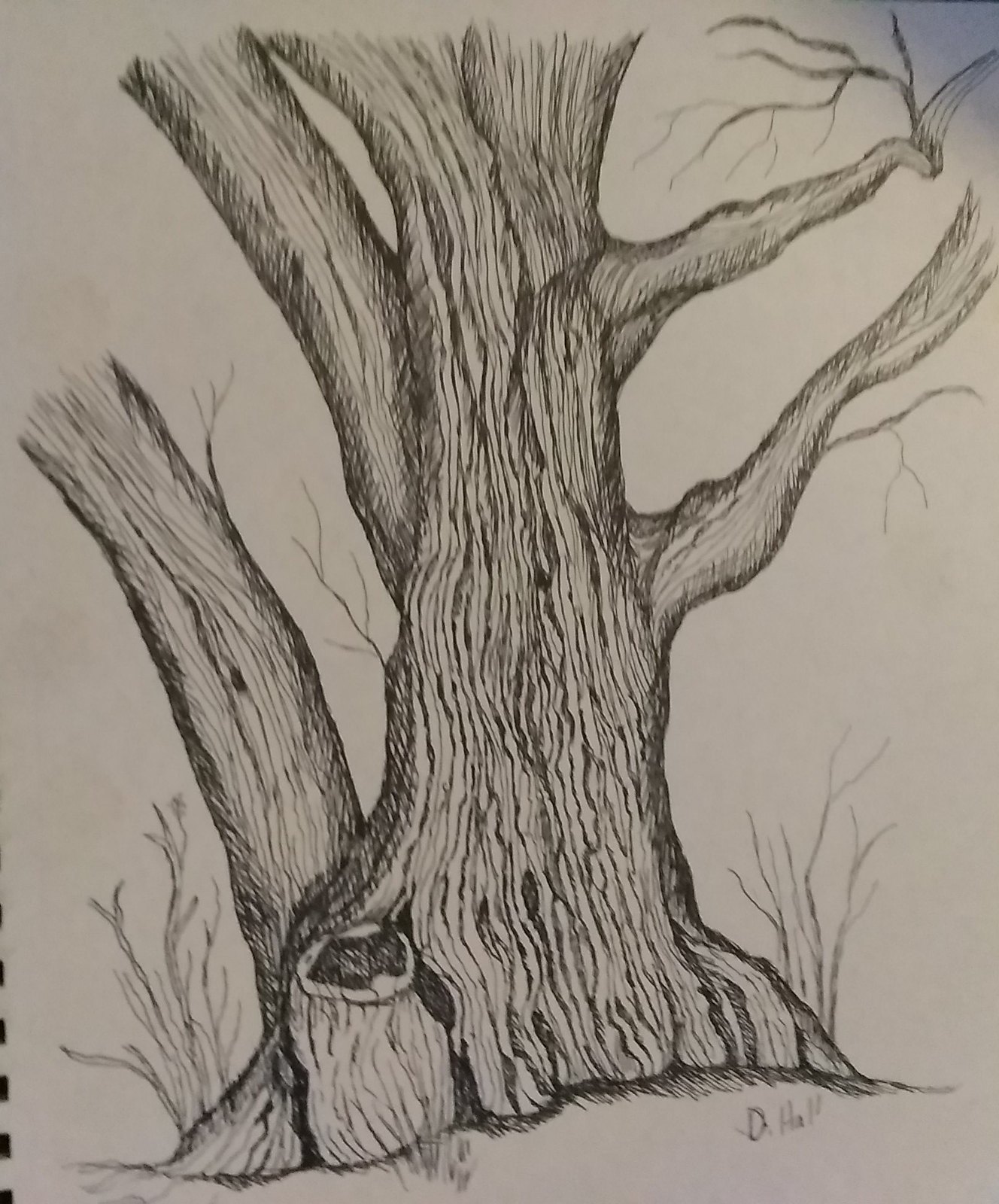In this detailed black and white sketch, an old, leafless tree stands prominently against a light gray backdrop, its gnarled trunk exhibiting rough, textured bark. The asymmetrical branches extend haphazardly—larger, more robust ones jutting out from the left side, while smaller, twig-like branches protrude from the right. One notable branch on the left appears to have been cut off cleanly at its base. The sparse, bleak nature of the tree evokes a winter scene, further emphasized by the bare ground surrounding it. In the background, additional trees or undergrowth rise subtly, hinting that the tree might be situated on a hillside, enhancing the somber and desolate atmosphere.